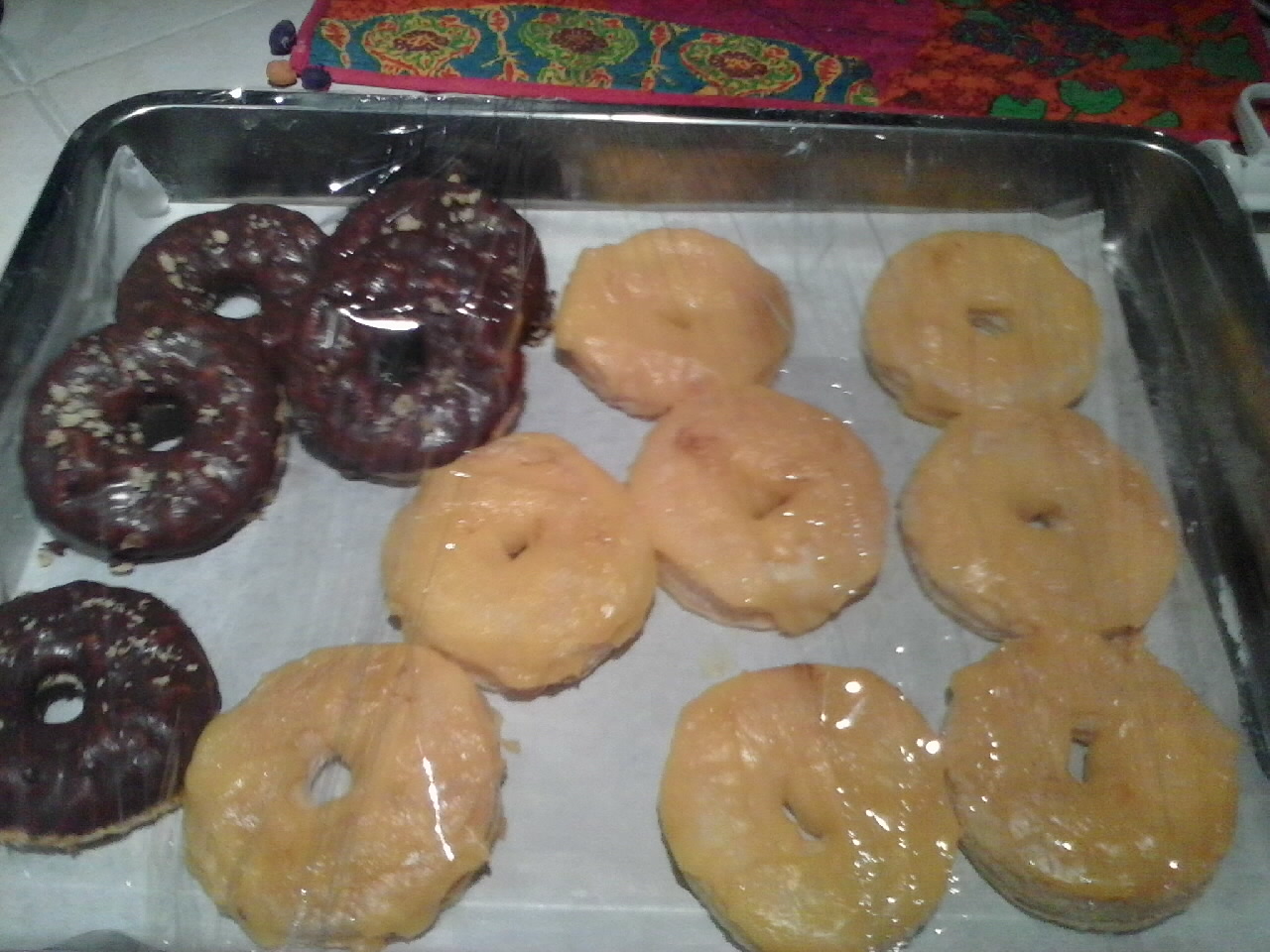This photograph features a baking pan sitting atop a counter or table, adorned with a sheet of parchment paper at the bottom. Inside the pan, at the left, there are five chocolate-glazed doughnuts, seemingly sprinkled with nuts or coconut. On the right side, there are eight plain, yellowy-cream-colored glazed doughnuts, both types covered with saran wrap. The baking pan is metallic and the entire setup reflects light from above, creating a slight glare on the cellophane. In the background, a brightly colored cloth with purple, red, green, yellow, and blue designs partially extends beyond the pan, contributing a vibrant contrast to the scene. There are no words or text visible in this image.